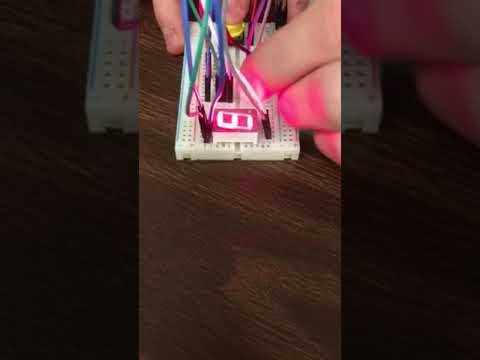The image is a close-up of a white circuit board being handled by a pair of Caucasian hands. One hand is positioned at the top, while the other shows only three fingers on the right. The circuit board features an intricate array of pin holes and several black jacks being plugged into various ports. Surrounding the circuit board are numerous wires in different colors including black, white, red, purple, and lighter blue, some of which extend off to the left. Above the hands, these colorful wires connect to the board, highlighting the complexity of the setup. The board is on a brown surface, and to the upper left, a small LED screen displays the number eight in a glowing light. The picture's framing and the subject matter suggest that it might be taken from an electrical engineering-themed video.